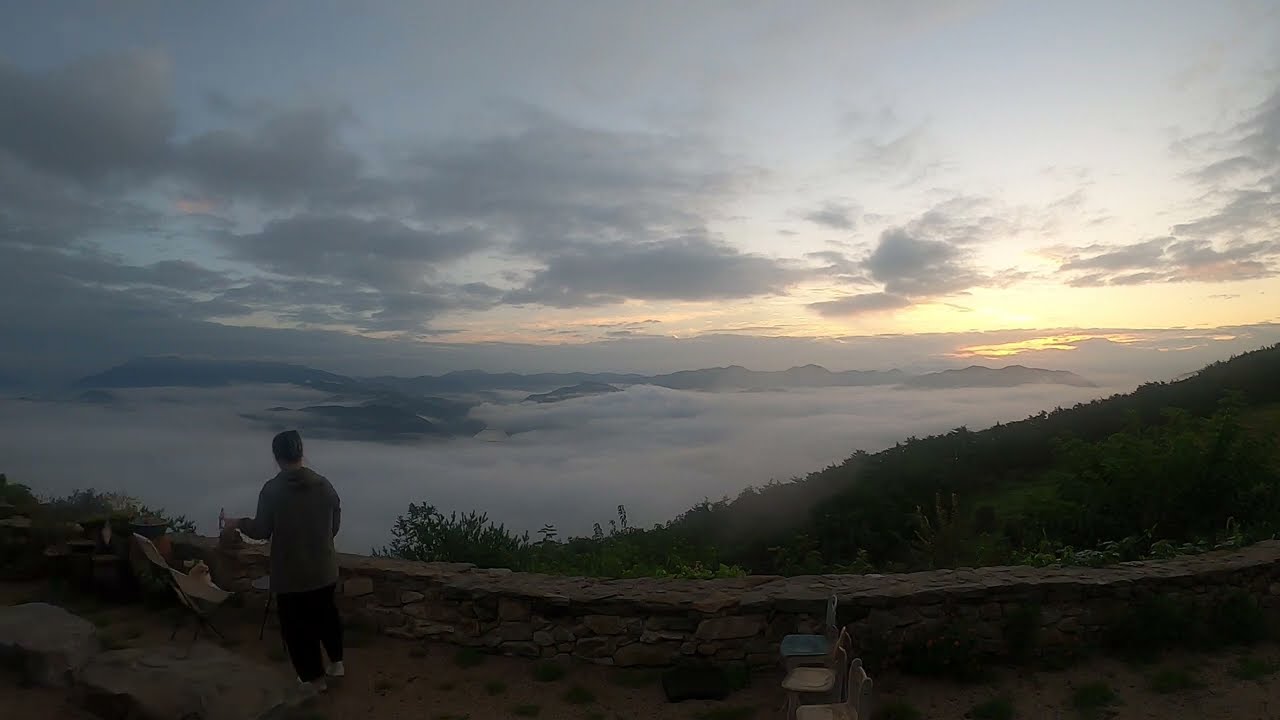Perched atop a mountain high above the clouds, the scene features a lone figure standing near the left side of a low, stone wall, almost knee-high, gazing down the steep hillside. The sky above is a canvas of dim, grey clouds tinged with the soft hues of an ethereal sunset, where occasional bursts of yellow and orange light peek through. Mist and fog envelop the surrounding peaks, offering an almost heavenly view below. The tranquil foreground is populated by three chairs lined up along a road in front of the wall, and nearby, a man appears to be walking, possibly pushing a baby carriage or carrying a basket. The overall atmosphere is serene and contemplative, capturing the majesty and peace of the mountain summit at dusk.